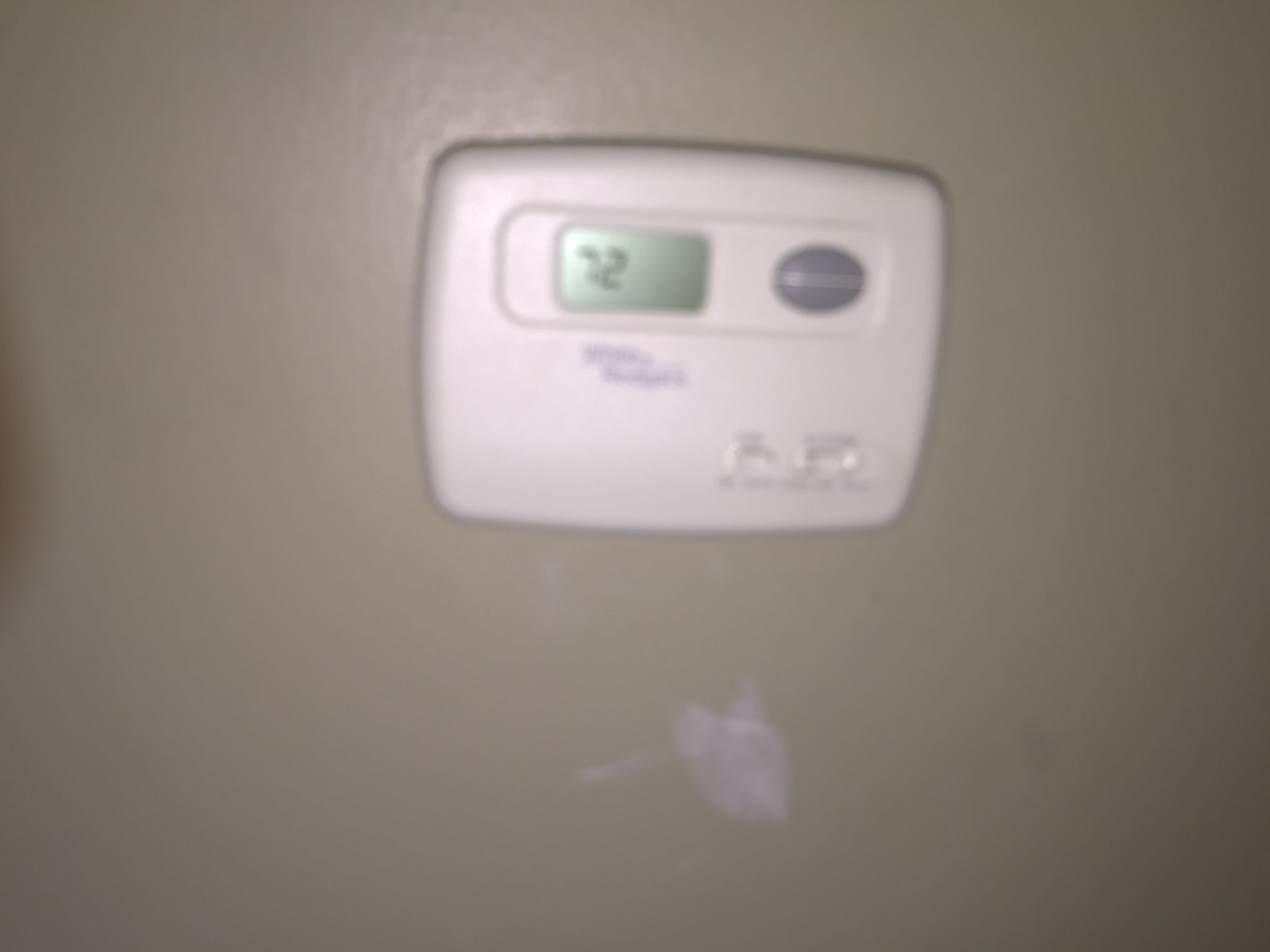This horizontal rectangular image, captured with a low-quality, likely smartphone camera, displays a blurry view of a wall featuring a basic thermostat. The thermostat reads "72 degrees" despite the blurriness obscuring finer details. Beneath the temperature display is an unreadable brand name, while to the right of the temperature is a similarly indecipherable gray area. The thermostat also includes two small switches at the bottom, though the poor image clarity makes it impossible to determine their labels or functions.